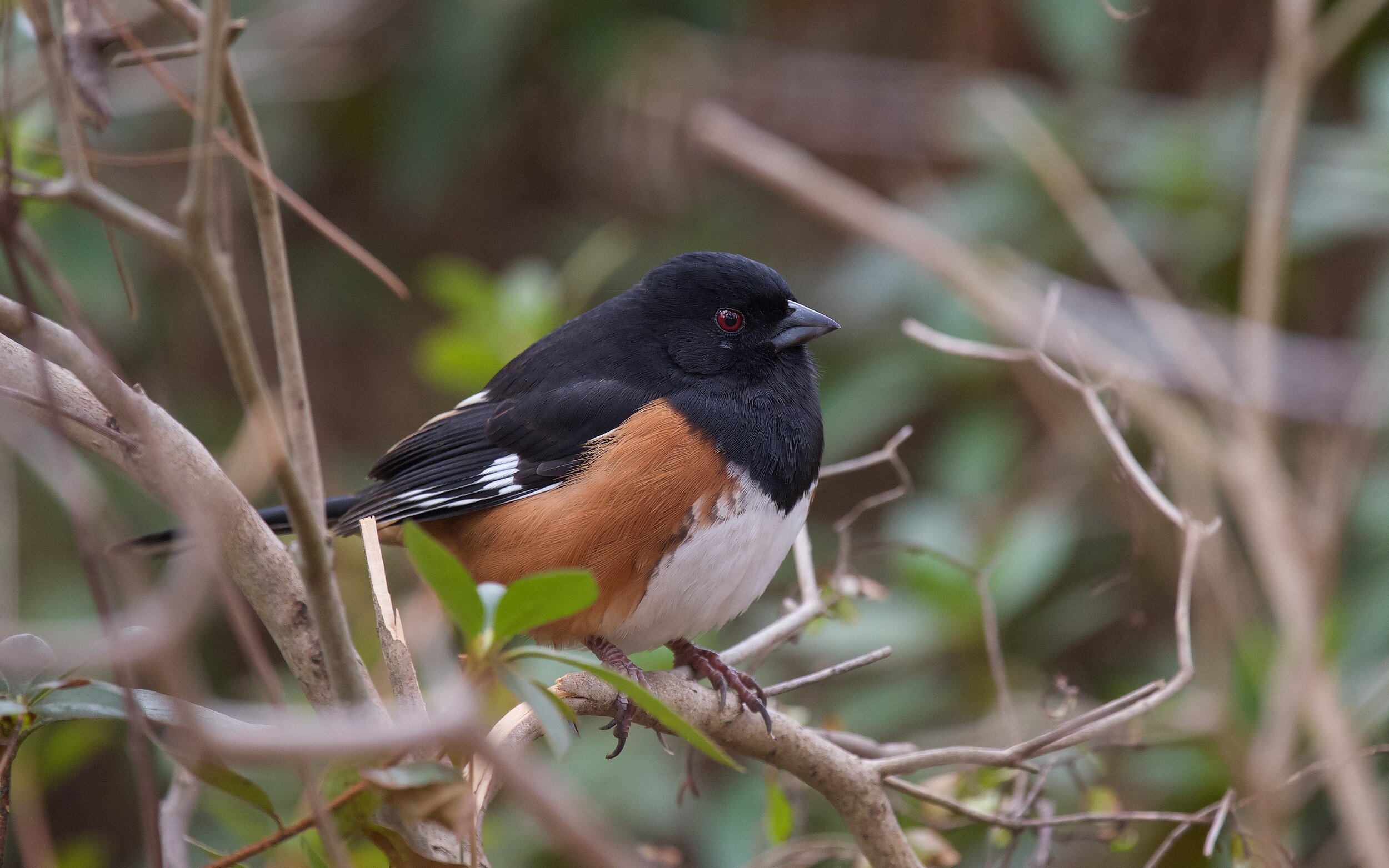This photo captures a small bird, perched on a branch with sparse foliage, likely during the fall or winter season. The bird appears to be a stout, possibly a finch or some type of cardinal, characterized by its distinct black crest that forms a sharp V shape on its breast. The bird's top half and head are black, extending down its back to its tail, with black and white wings. Its breast is a crisp white, transitioning to a light reddish-brown on the sides and lower part of its body, giving a fawn-like appearance. The bird has dark red, almost brown eyes and a short, stubby black beak. The background of the image is intentionally blurred, focusing the viewer's attention solely on the bird and its branch, highlighting the wildlife aspect of the scene.